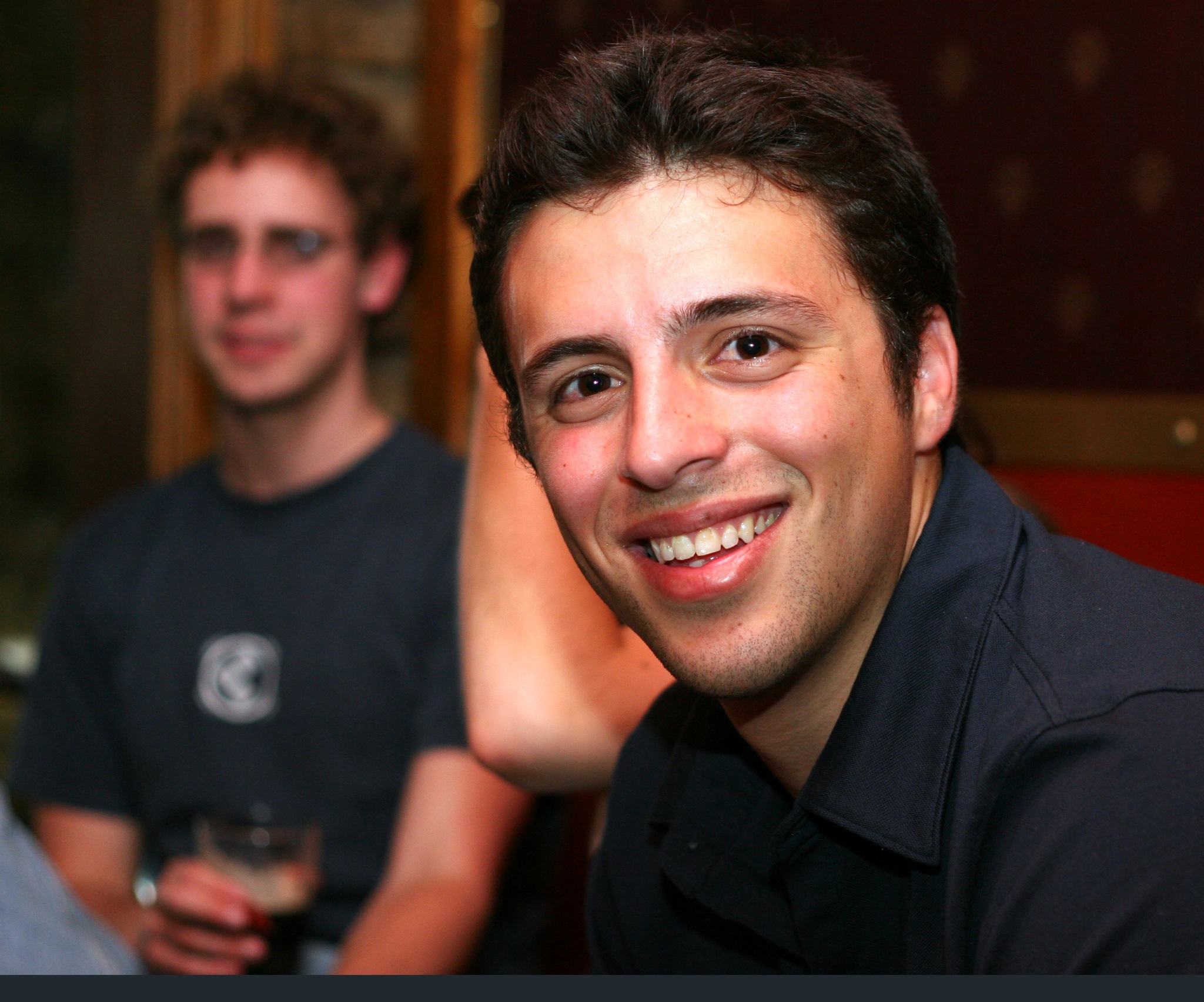The photograph captures two Caucasian men in what appears to be a bar or restaurant setting. The man in the foreground, who is clear and prominently featured, is smiling broadly and looking directly into the camera. He has short, dark brown hair, brown eyes, and is clean-shaven, sporting a dark blue or black polo shirt. His white, straight teeth are visible as he grins. To his left and slightly behind him, there is another man whose image is more blurred. This man has short, curly brown hair and wears glasses that transition from clear to sunglass-like tint in the light. He is also dressed in a dark shirt and appears to hold a glass of a dark beverage, possibly soda or stout beer, in his right hand. Behind them, the setting includes elements of the restaurant or bar, such as a red wall and brown wood framing. The overall color palette of the image includes shades of dark blue, brown, tan, red, and black.